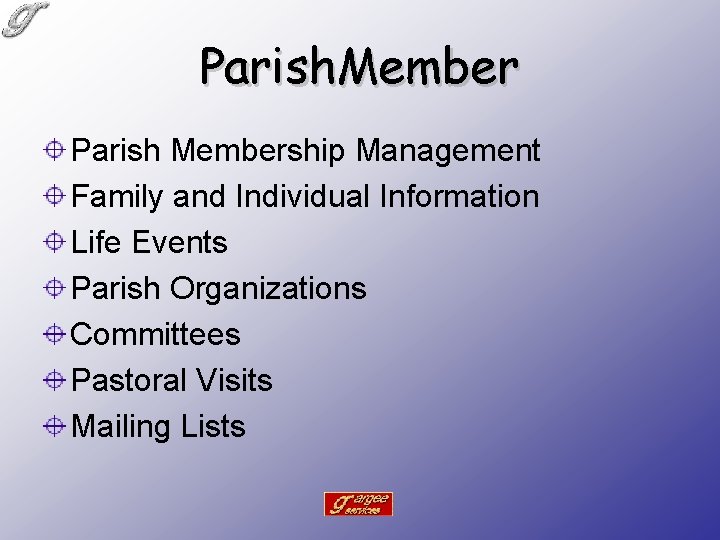The image is a digitally created slide, likely from a slideshow presentation. It is rectangular in shape, measuring approximately six inches wide by four to five inches tall. The background features a gradient that transitions from a deep purplish-blue in the lower right corner to a very light, almost pale blue in the upper left corner. In the upper left corner, there's a lowercase cursive letter "g" written in silver or gray. 

At the top center, the words "Parish Member" are prominently displayed in black print, with no space between "Parish" and "Member" but with both the "P" and "M" capitalized. Below this title, aligned vertically along the left side, are several bullet points marked by purple circles with a black cross in the center, resembling a scope. The text next to each bullet point is also in black and reads as follows: "Parish Membership Management," "Family and Individual Information," "Life Events," "Parish Organizations," "Committees," "Pastoral Visits," and "Mailing Lists."

At the bottom center of the slide, there's a red rectangle with a white outline, containing a stylized yellow "G" followed by the word "ARGE," possibly part of the phrase "Gargi Services." This combination of colors and detailed layout creates a visually informative slide focused on parish member management and related information.